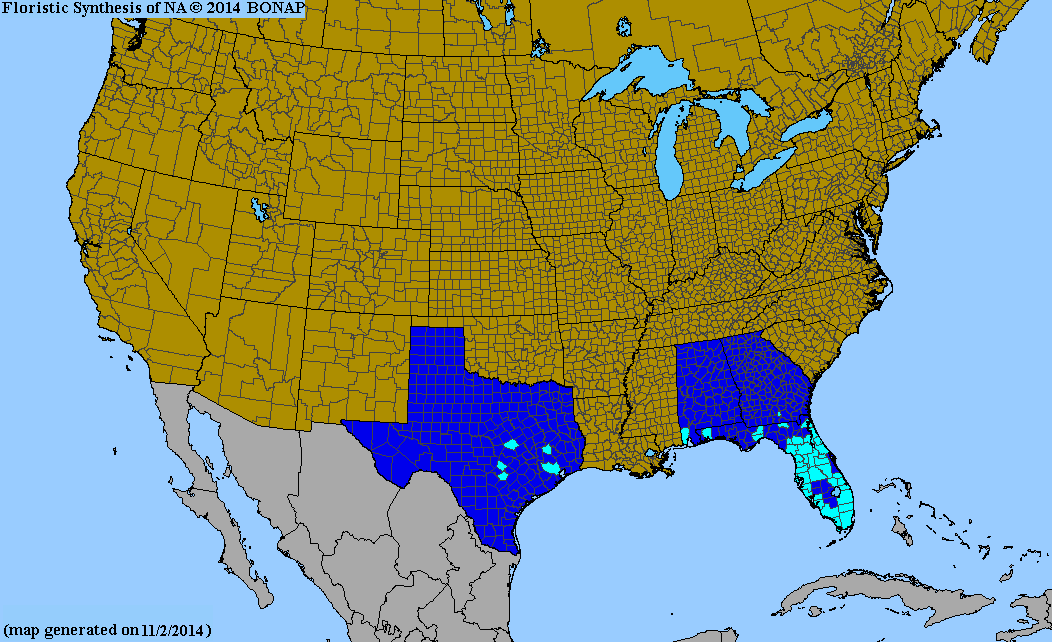This image is an artistic map of the United States, showcasing each state with distinctive county lines. Most states are depicted in a mustard yellow color with black grid-like outlines indicating the individual counties. Texas and Florida are prominently highlighted in dark blue, with sections within the states shown in lighter blue shades. Additionally, Arkansas, Georgia, and Alabama are also presented in blue hues. The map includes parts of neighboring Mexico in a gray tone and some Canadian provinces also in mustard yellow. The surrounding waters, including the Atlantic, Pacific, and the Great Lakes, are portrayed in a teal color. In the upper left corner, black text reads “Floristic Synthesis of NA, 2014, Bonap,” and in the lower left, the caption “Map Generated on 11-2-2014” is noted, indicating the date of generation.